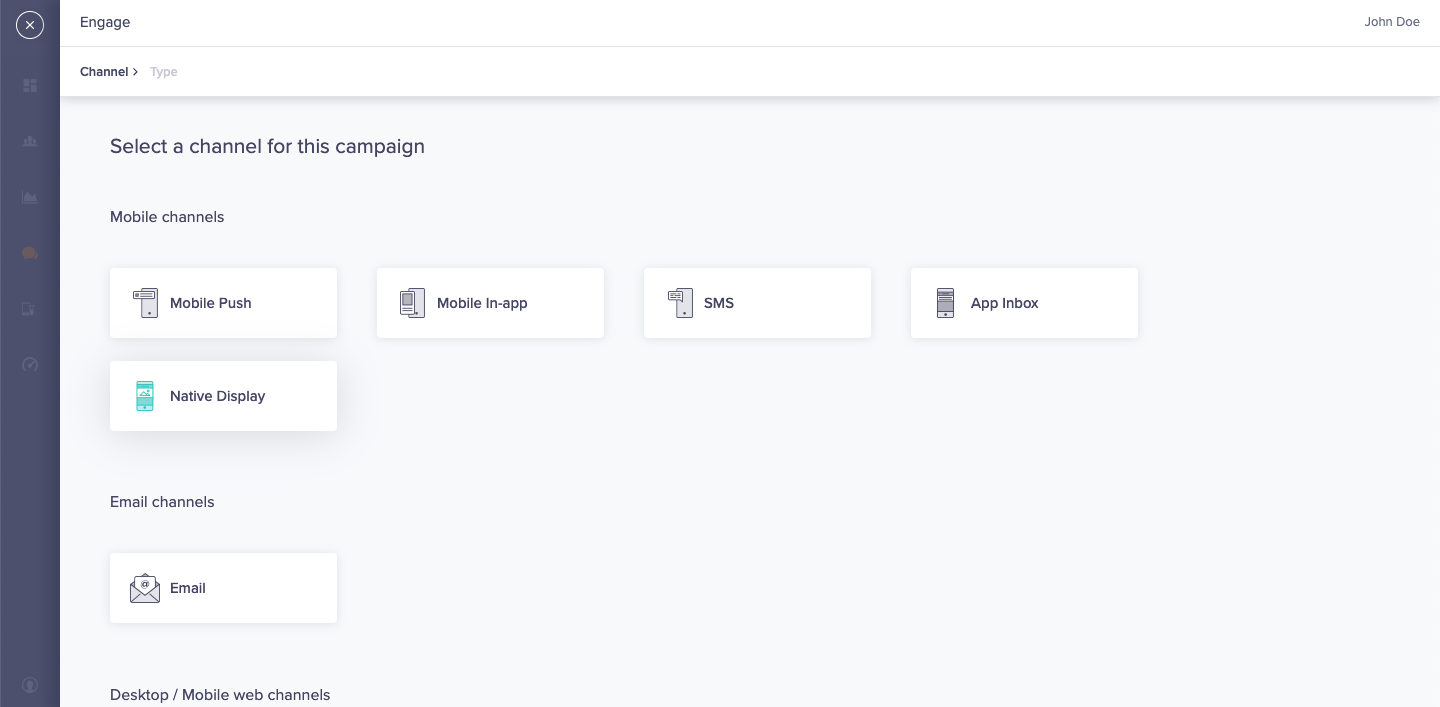The image depicts a monochromatic, minimally designed webpage from a website with the header "Engage" located in the upper left corner. The top of the page features a black bar with a white circle containing an 'X' on the left side. Directly underneath is a white bar labeled "Channel," with a prompt to type on the right side. On the upper right corner, the name "John Doe" is displayed next to an icon.

Below the header section, the page instructs users to "Select a channel for this campaign." The following sections are categorized into "Mobile Channels," "Email Channels," and "Desktop & Mobile Web Channels."

In the "Mobile Channels" category, several options are presented in gray boxes with icons on the left side, including:
- Mobile Push
- Native Display
- Mobile In-App
- SMS
- App Inbox

In the "Email Channels" category, a gray box labeled "Email" is also present with an accompanying icon on the left.

The background of the page is predominantly gray, with all selectable options encased in slightly darker gray boxes. There is a vertical black bar running along the left side of the page. The website's overall design is simple and monochromatic, using shades of black, white, and gray. The minimalistic icons blend into the background, resulting in a very plain and unexciting visual appearance.